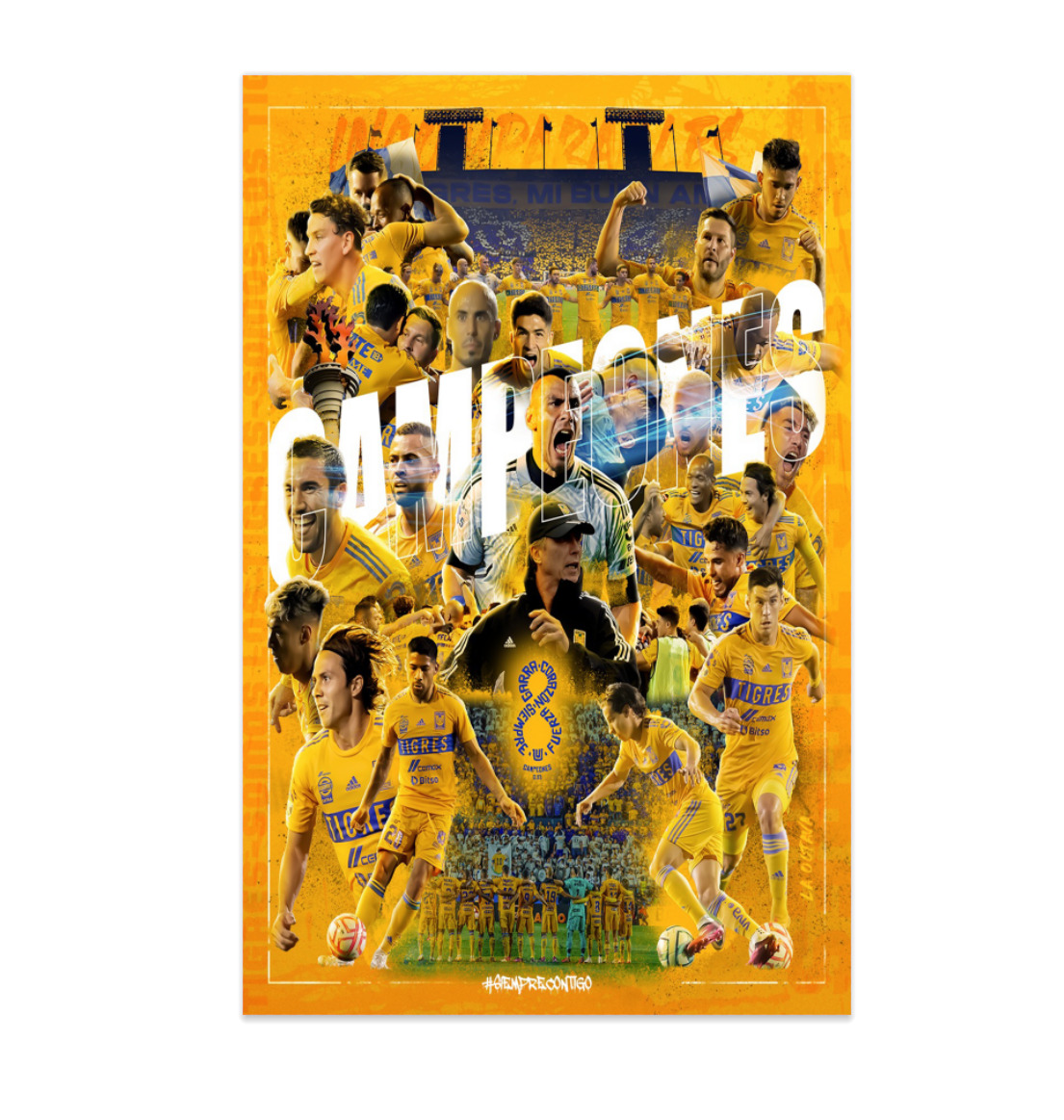The image is a vertically rectangular, full-color digital print piece that resembles a magazine cover or a team poster with a slightly orangeish background. It depicts the jubilant celebration of soccer players from the team "Tigres," dressed predominantly in yellow uniforms with blue text and highlights. The players are seen cheering, hugging, and displaying various emotions of triumph, with some holding soccer balls, indicating victory. The text "campeones," which means "champions," is written in white, though partially obscured by the players' heads.

The central focus is on two distinct players: one in a white top, possibly the goalkeeper, with a black shirt underneath, and another in a black or dark blue uniform, potentially a referee or coach. The individual with the white top has a wide-open mouth and a striking mohawk hairstyle, adding dramatic flair to the scene. The background features a digitally enhanced image of stadium stands filled with cheering fans, many dressed in yellow, amplifying the celebratory atmosphere. The players' yellow socks are detailed with black and white stripes, adding to the uniformity and vibrancy of the team's attire.